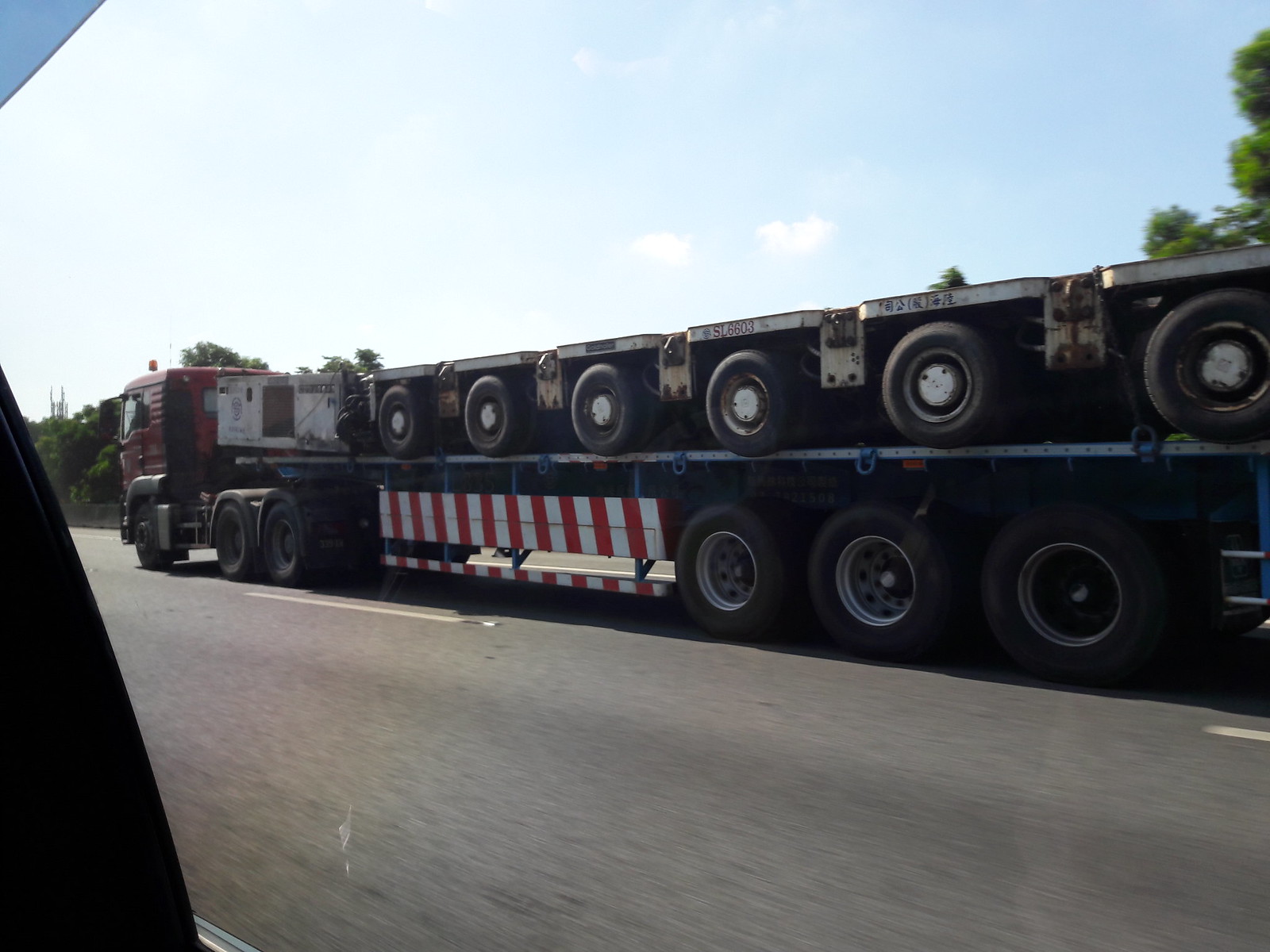The photograph captures a red semi-truck pulling a red and black flatbed trailer down a multi-lane asphalt highway. The trailer is hauling a series of equipment that appear to be dark boxes, each with a tire mounted on its outer edge, resembling small carts or mining carts. The trailer features a red and white striped mud shield along its side. The image, taken on a bright, clear day with a blue sky dotted with scattered white fluffy clouds, also shows some green trees in the background. The road appears slightly blurry, suggesting motion. There are additional color details: a small triangle of blue in the upper left-hand corner and a large triangle of black in the lower right-hand corner. The photo was likely taken from inside another vehicle.